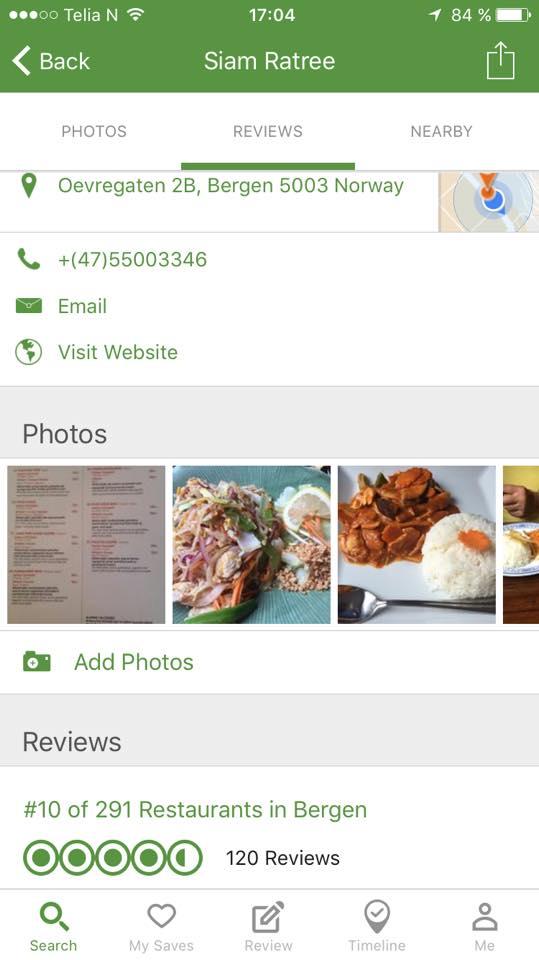This image, captured from a smartphone, showcases the user interface of a restaurant-related app. At the top, a green bar prominently displays essential device information, including the current time and battery status. Directly beneath this bar, the name "Siam Ratree" is featured in bold white letters, marking the identity of the restaurant.

Beneath the restaurant name, three navigational tabs are available: "Photos" on the left, "Reviews" in the center, and "Nearby" on the right. The "Reviews" tab is currently selected, providing detailed information about the restaurant. Below the tabs, important contact details are presented on a white background, including the restaurant’s address, telephone number, email, and a link to its website.

The main content area features a photo slider, which users can scroll through horizontally. The visible images include a menu, two food items, and a partially visible fourth image depicting a plate of food alongside a hand and wrist clad in a black jacket.

Moving further down, there's an option to add photos, followed by a reviews section. Text in green letters indicates that the restaurant ranks number 10 out of 291 restaurants in Bergen, Norway. The establishment has garnered 120 reviews and boasts a high rating of 4.5 circles. At the bottom of the screen, five interactive icons are arranged from left to right: "Search," "My Saves," "Review," "Timeline," and "Me," providing further navigational options for the user.